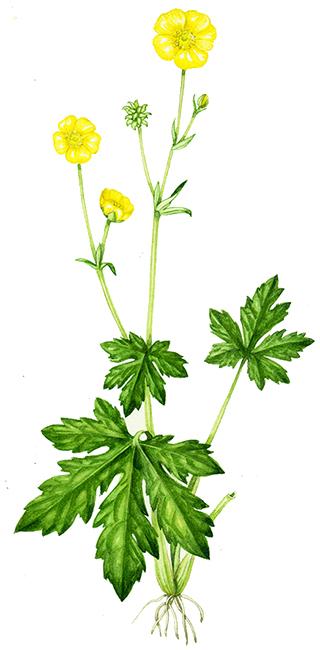This is a detailed illustration of a ranunculus, showcasing the entire plant from its vibrant yellow flowers at the top to its roots at the bottom, all set against a solid white background. The yellow asteraceae-type petals, shiny and outward-facing, give a summery appearance to the flowers. The stems are a light green and rather thin, supporting the palm-like leaves, which consist of five parts emanating from a central point. These leaves appear well-manicured and healthy. Towards the top, the illustration highlights the flowers in various stages: three fully bloomed with five yellow petals and several bulbs that are about to bloom. The roots are depicted as a light, almost whitish green and are relatively short. The artist's skillful shading and coloring bring a sense of realism and simplicity to this summery floral piece.